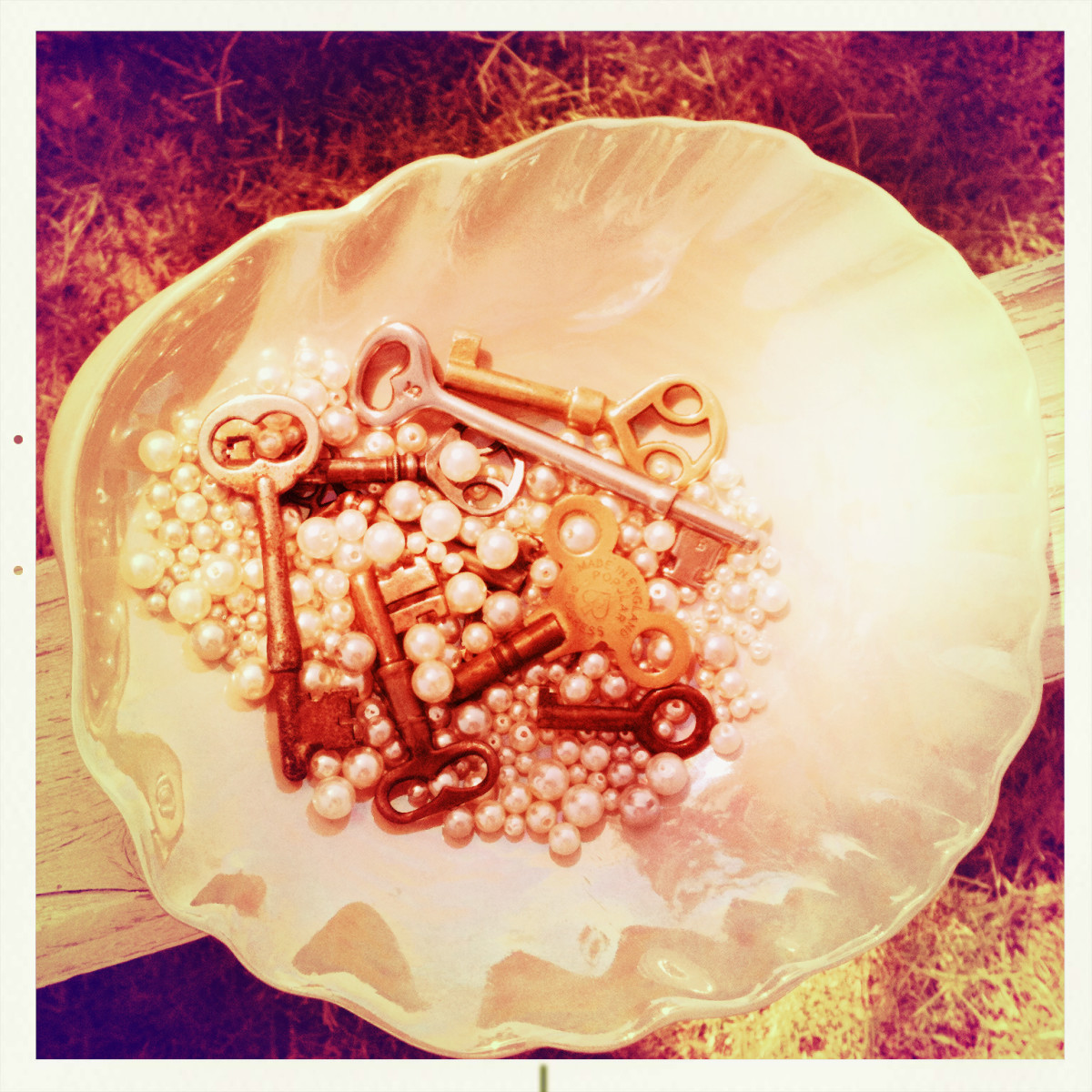The image is a detailed photograph of a large, shiny white seashell, either naturally white or painted with reflective enamel. The seashell, which is resembling a dish, lies on a board and holds a collection of intriguing items. Inside the shell, there are various white pearls of different sizes, some suitable for beading, interspersed amongst a set of old-fashioned keys. These keys, numbering around six, are in various states and colors including gold, bronze, rusty, and silver, and appear to be the types once used for clocks or doors. The background of the image is a striking red, with a grungy, meshy texture that almost evokes the appearance of flames. There is also dried grass scattered in the background, adding to the rustic, aquatic theme of the composition.